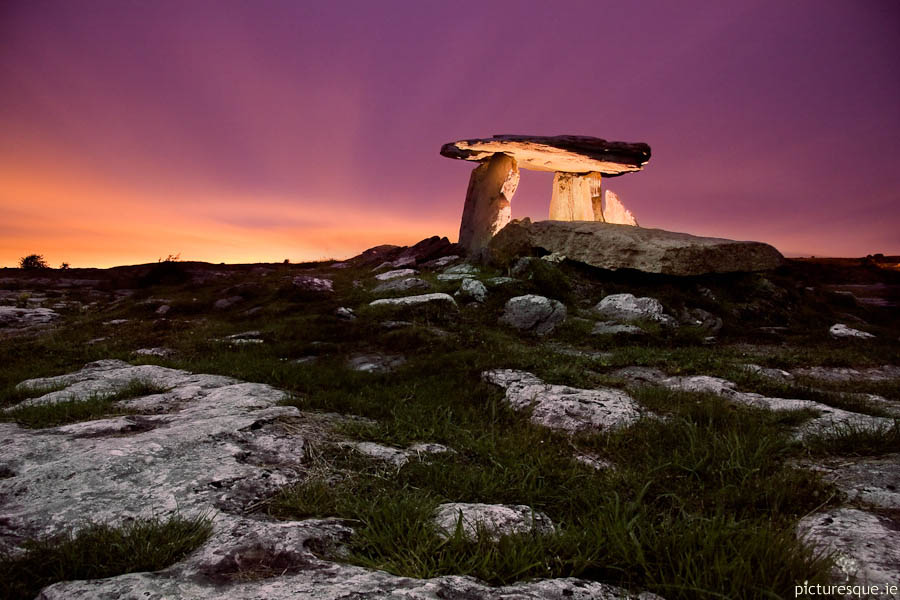In this captivating image reminiscent of Stonehenge, the rocky foreground is interspersed with patches of resilient grass. The focal point is a striking stone formation: two tall slabs standing upright, supporting a massive horizontal slab that forms a primitive arch. This ancient structure stands majestically illuminated by the setting sun, which casts a golden glow that transitions through a warm peach hue into a rich purple sky. The horizon showcases a brilliant yellow-white area blending seamlessly into the purples, enhancing the ethereal quality of the twilight. The ground around the rock formation is strewn with various-sized stones, creating a sense of ancient ruins in a solitary, treeless field. The serene and untouched nature depicted gives the scene a timeless beauty, further accentuated by the caption "picturesque.ie" subtly placed in the bottom right corner. This evocative image captures the haunting beauty of nature and ancient architecture bathed in the magical light of sunset.